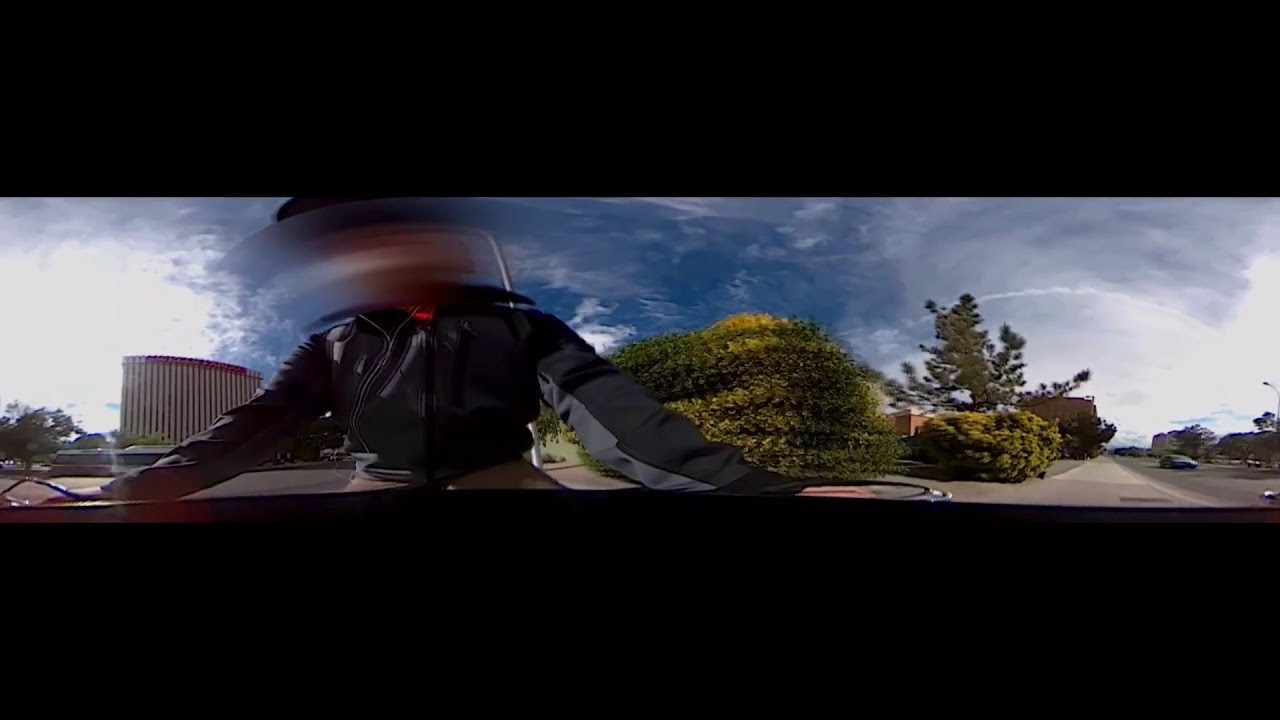The image features a horizontally rectangular, somewhat blurred photo with prominent black bars on the top and bottom, creating a narrow and wide frame of the scene. At the center, there's a person whose head is blurred, possibly for privacy reasons. They appear to be wearing a dark gray or black jacket with gray accents on the inner parts of the arms, and tan pants. Their arms are outstretched as if holding the handlebars of a bike or motorcycle, although the black bars obscure the hands and handlebars. It seems they might also be wearing a dark cap.

The background reveals a partly cloudy sky, with a mix of gray and white clouds against patches of blue. On the right side, there are tall green shrubs and some green trees. The left side features more green shrubs and trees, a grayish concrete building, and a large white building in the left-hand corner. Additionally, the scene includes elements of a roadway, a sidewalk, and a visible car, indicating an urban setting. The overall image appears slightly distorted, giving the impression that parts of the background, like the bushes and sky, are stretched unnaturally.